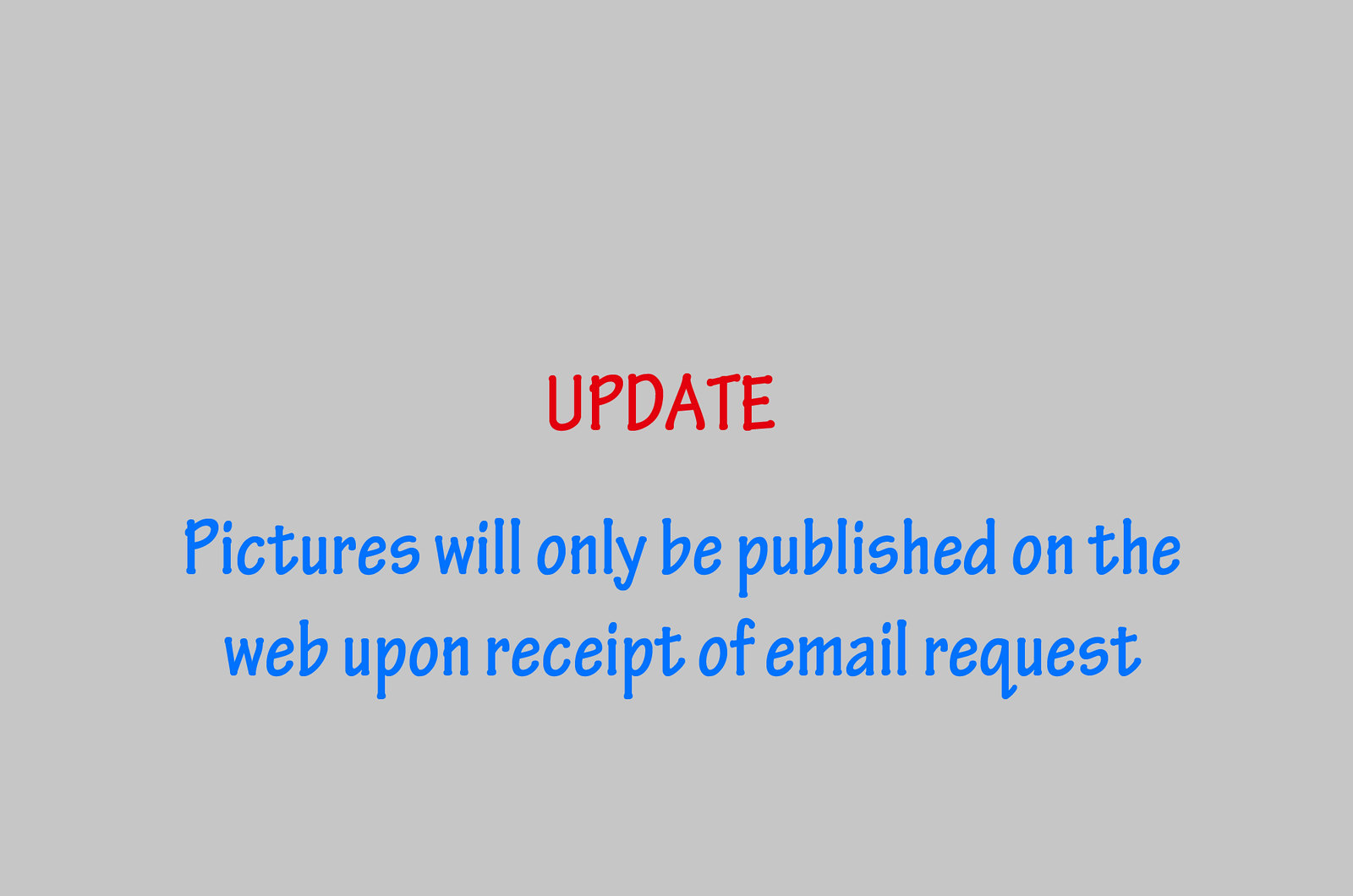The image is a horizontally oriented light gray rectangle with uniform color, featuring centered text. At the top center, in all caps red letters, the word "UPDATE" is prominently displayed. Below this, in blue letters, it reads: "Pictures will only be published on the web upon receipt of email request," with only the 'P' in "Pictures" capitalized and no punctuation at the end. The text is the sole content on the image with no borders, lines, or decorations.